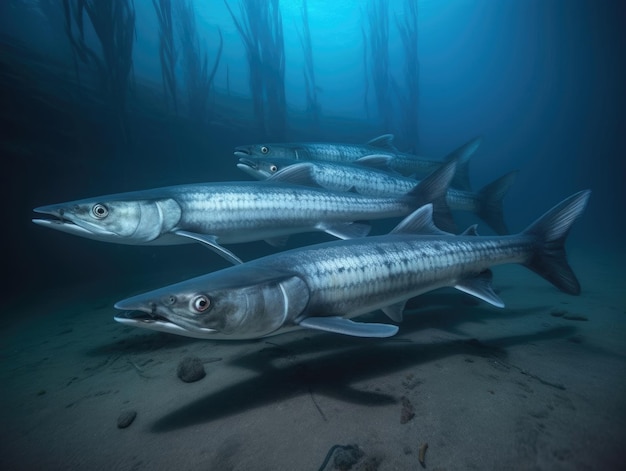At the bottom of the sea, a scene unfolds featuring four long, slender, silver-gray fish with defined scales, swimming in a westward direction. Positioned centrally, these fish span from approximately 30% to 60% up the image, moving at roughly the 7 or 8 o'clock position. They hover close to the dark, sandy ground which is littered with a few scattered rocks. Behind them, tall stalks of silhouetted seagrass rise up, creating a shadowed backdrop. Sunlight penetrates the murky, dark gray waters from above, casting shadows of the fish onto the sea floor and illuminating the scene, making it appear both strikingly realistic and possibly a highly rendered digital artwork.